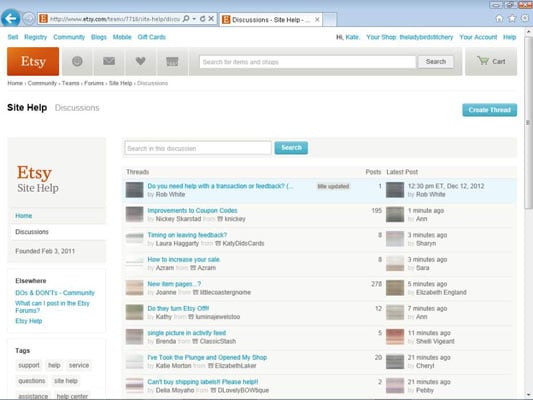The screenshot captures a webpage viewed in a web browser, specifically from Etsy.com, a popular online marketplace for handcrafted and vintage items. The image is of low resolution, making the finer details difficult to discern. The browser displays only one tab, which is opened to the Etsy help section. This section appears to be a discussion board where users share and seek advice on various topics related to selling on the platform. Visible posts likely include questions about boosting sales, optimizing coupon codes, and managing feedback timing. The overall context suggests that the users are primarily small-scale, self-employed crafters seeking to enhance their online shops.